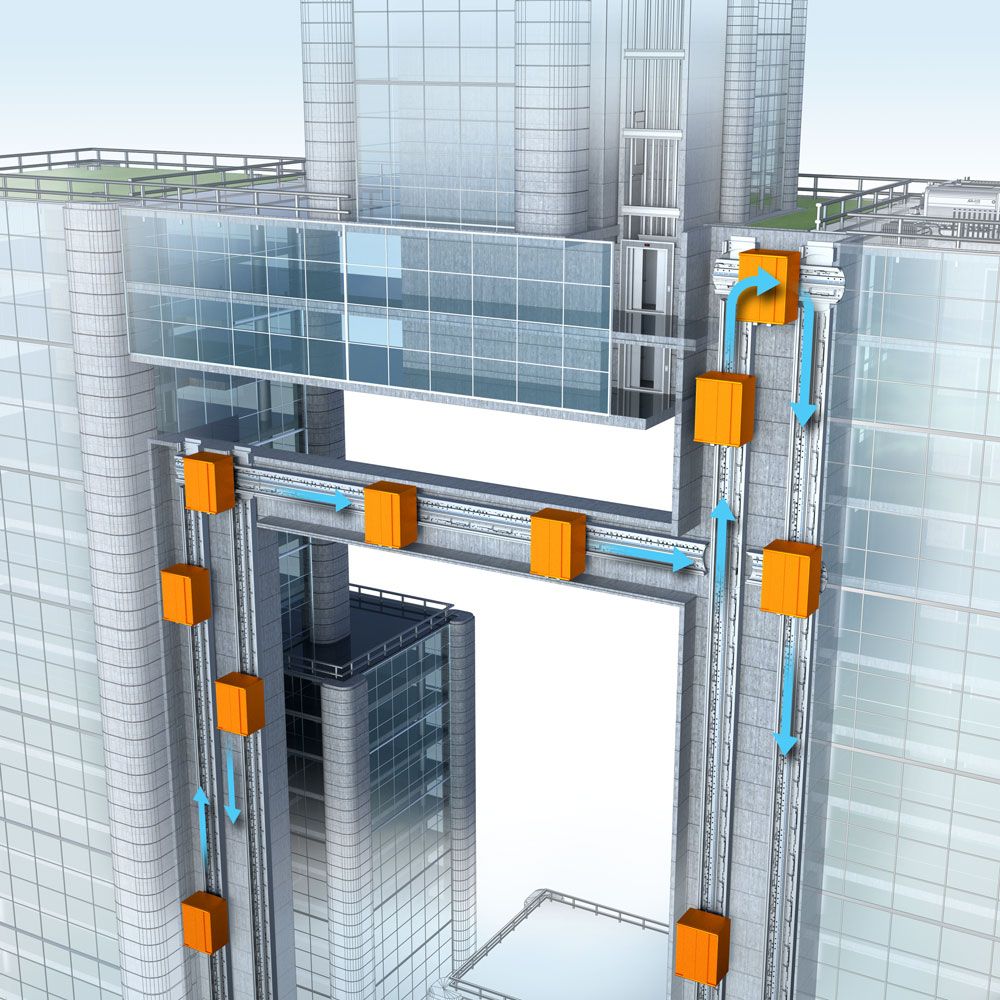The image depicts a digitally-created architectural model of a towering skyscraper featuring an advanced, innovative transport system. The building is characterized by its multi-leveled structure with numerous windows and is composed of rectangular prism shapes on either side. At the top, an additional rectangular prism projects upward from the center. There are pathways that visually connect the two main vertical sections of the building, suggesting possible walkways or linking structures. However, the focus is on a unique elevator system, outlined with cubes of orange and directional arrows, indicating vertical and horizontal movement capabilities. The elevators are positioned externally, akin to the design seen at the Rio Las Vegas Casino. The image implies that these elevators can travel up, down, and sideways, providing an inventive method of transporting individuals between different parts of the skyscraper, highlighting a cutting-edge approach to urban transport infrastructure.